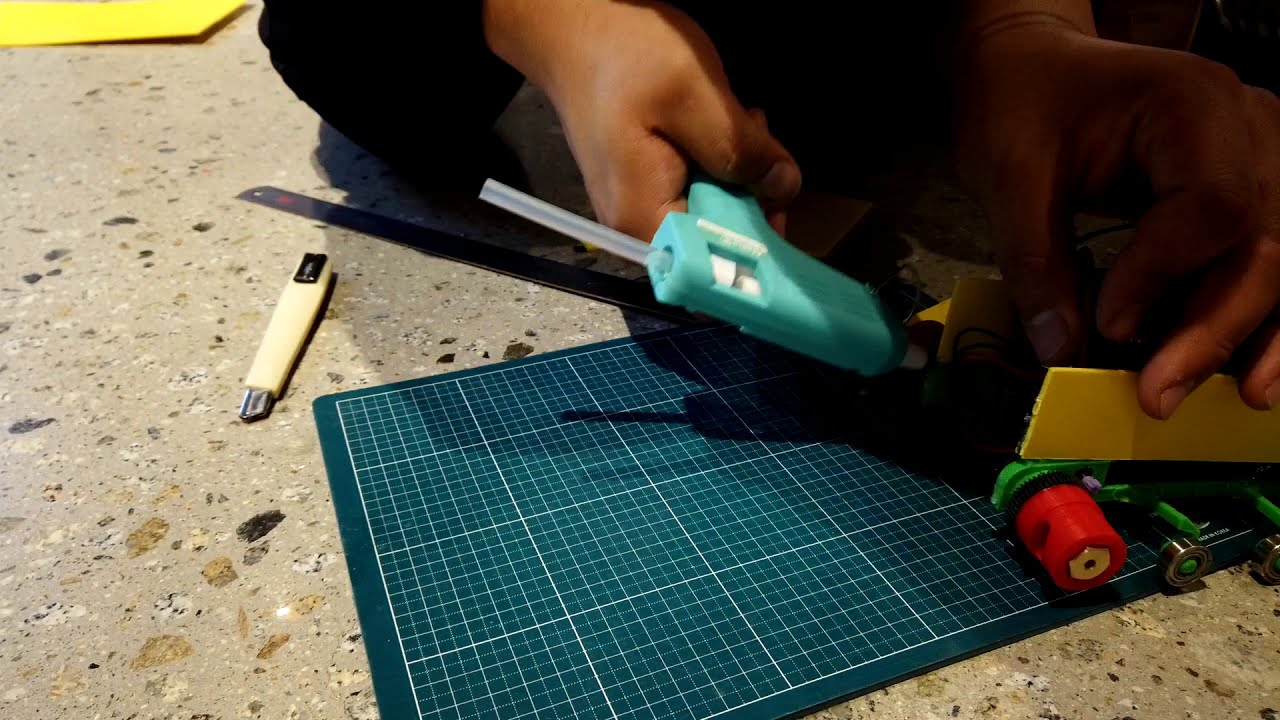In this highly detailed color photograph, oriented in landscape, a person with dark skin tone is engrossed in a meticulous craft project, seated on a light beige, speckled marble-patterned floor. Only their hands and knees are visible, as they skillfully use a bright aqua hot glue gun in their right hand to affix components on a dark green craft mat marked with a white grid pattern. In their left hand, they hold a yellow, ruler-shaped piece. Nearby on the mat lies a beige-handled craft knife. Scattered about are vivid components in yellow, red, and green, possibly part of a complex, unidentifiable structure. A piece of yellow paper peeks into the frame from the top left corner, and additional crafting tools, including a ruler, subtly enhance the scene. The person's focus and the detailed assembly of materials suggest a blend of precision and creativity in their work.